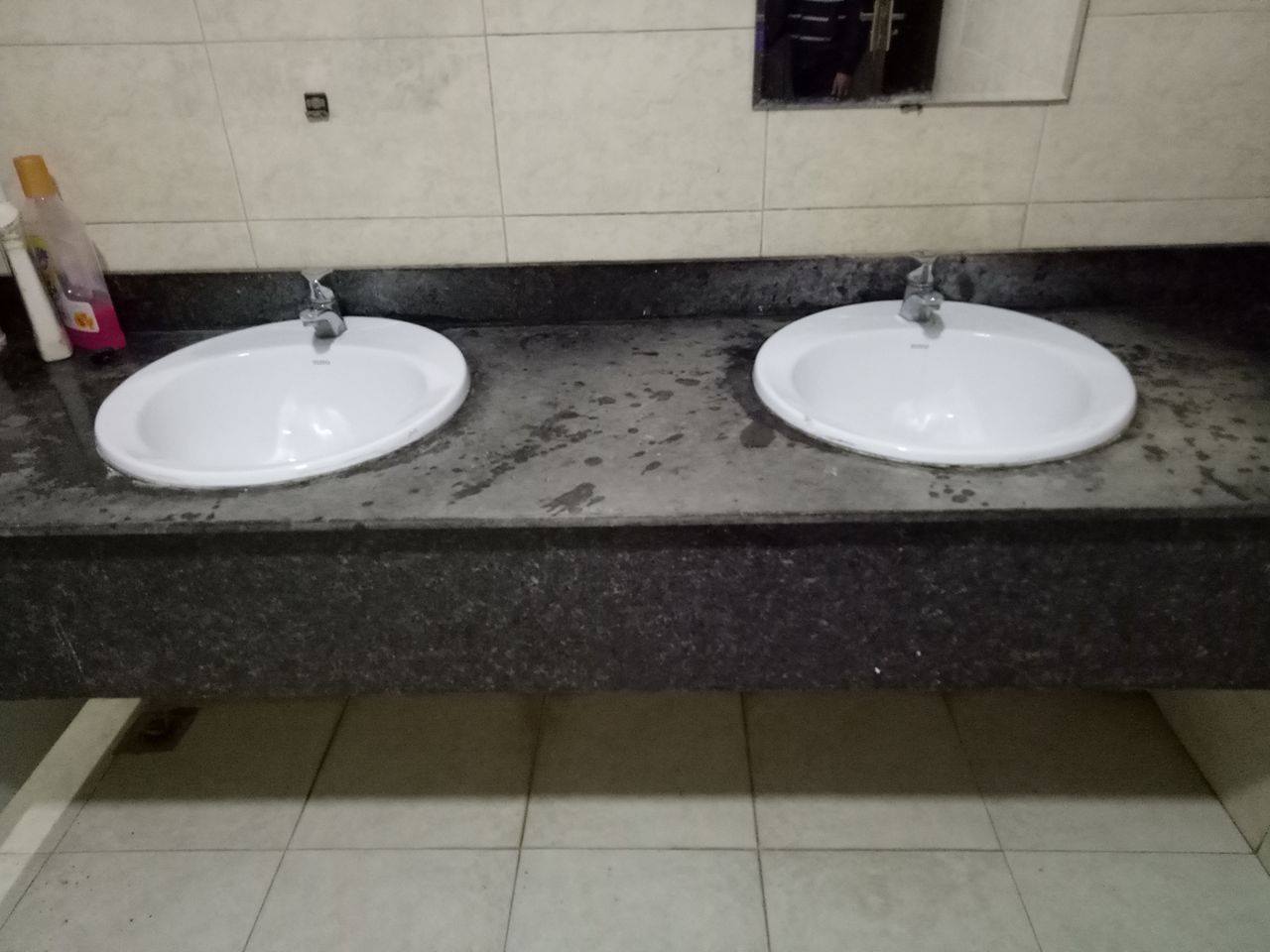The image depicts a section of a public restroom featuring a pair of bright white porcelain sinks with silver single-handle faucets, set into a black countertop that appears to be marble or granite with gray veining. The countertop, which looks somewhat dusty, stretches beneath a large mirror directly above the right sink, reflecting part of a person's lower body, hand, and shirt. The floor is covered in gray tile that seems somewhat dirty, while the wall behind the sinks is adorned with clean, white tiles. On the left side of the countertop, there are two bottles—one appears to be a purple soap dispenser, and the other is a white, opaque bottle. Additionally, there is an empty clasp mounted above the left sink, suggesting a space where a mirror might once have hung.